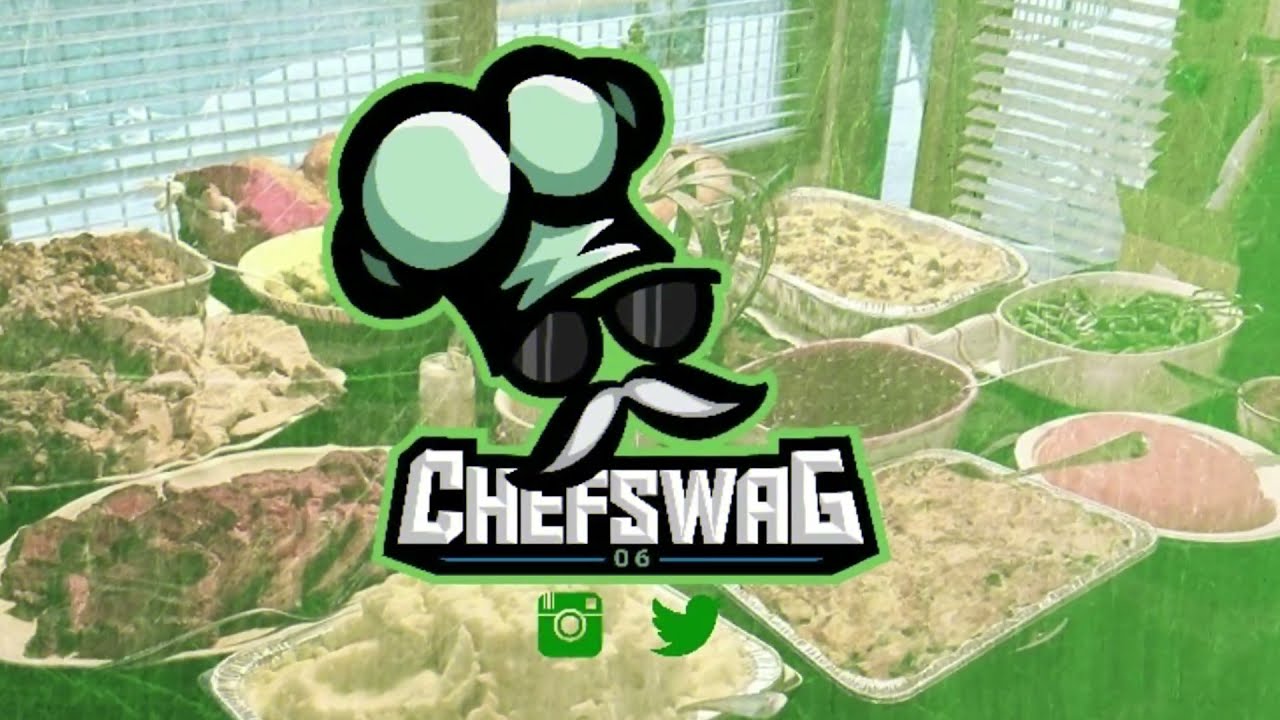This image, likely a screenshot, showcases an indoor setting that appears to be a kitchen or a restaurant with an all-you-can-eat buffet. The central focus is a logo featuring an animated face with black sunglasses and a long white mustache, topped with a mint green chef's hat. Below the logo, the text "Chef Swag 06" is prominently displayed in white letters. The logo is surrounded by small green icons of a camera and a bird, possibly indicating social media elements.

The backdrop is a table covered in a green cloth, laden with various food items, suggesting a Thanksgiving feast. The spread includes disposable aluminum foil trays and casserole dishes filled with mashed potatoes, stuffing, cranberry relish, green beans, carved turkey, roast beef, and other diverse dishes. The assortment also features a pinkish gelatin dessert, vegetables like beans, and a casserole with ground meat.

The top part of the image shows windows with venetian blinds, permitting outdoor light to filter in. The image palette is dominated by light green overlay, combined with hues of blue, white, gray, pink, red, brown, yellow, and light blue, adding a colorful yet slightly blurred aesthetic. Overall, the scene evokes the atmosphere of a festive food advertisement.